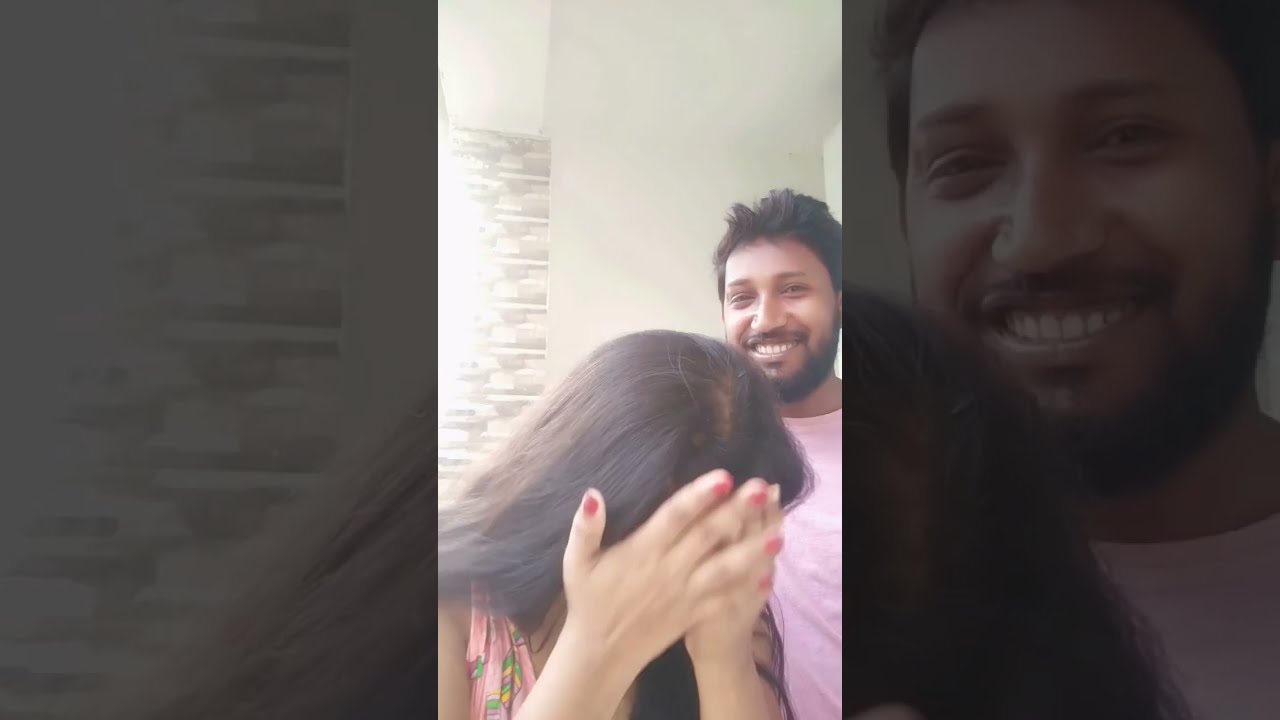This is a horizontally rectangular, borderless, three-panel image. The central panel is a vertically rectangular photograph depicting a man and woman indoors, with light streaming through a window, against a light gray wall that transitions into a patterned gray on the left. The central image is smaller and partially overlays two larger, darker-tinted close-ups of the same scene on either side.

The woman, positioned foremost in the central panel, has long dark brown hair and is wearing a pink top with a leafy design in shades of green, yellow, and pink. Her face is obscured as she covers it with her hands, which are adorned with pink nail polish, though they appear slightly blurry. 

Behind her to the right is a smiling man with brown skin, dark hair, a beard, and a mustache. He is looking at the camera and is also wearing a pink shirt. The left close-up primarily features parts of the woman's hair, while the right close-up focuses on the man's face.